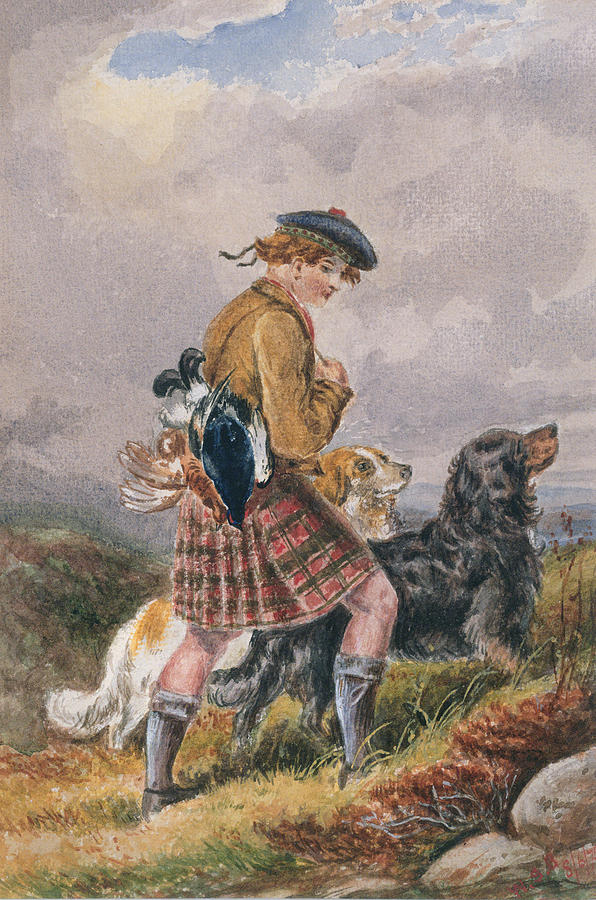This detailed portrait-oriented oil painting captures a young male in traditional Scottish attire, immersed in a hunting scene amidst a vibrant outdoor setting. His attire includes a long-sleeve tan jacket and a red and brown pleated kilt extending just above his knees. A blue beret with a red top graces his head, complementing his flowing red hair. His black socks fold over about three inches below his knees, and he wears shoes suitable for the rugged terrain.

The subject is depicted walking uphill, suggesting a sense of movement and purpose. He appears to be looking slightly downward to his right, concentrating on the path or his surroundings. Draped over his shoulder are two freshly killed birds, secured with a rope, indicating a successful hunting expedition. Accompanying him are two dogs: one predominantly black with tan markings, and the other mainly white with tan spots.

The setting is richly detailed with green and yellow grasses interspersed with patches of brown, indicating the changing seasons or varying vegetation. The landscape features rolling hills and distant mountains, presented under a sky filled with a mix of white and gray clouds allowing occasional sunlight to peek through. Stones dot the lower right corner of the painting, adding to the realistic texture of the terrain. The overall scene is bathed in daylight but framed by a heavily clouded sky, creating a balanced and immersive depiction of a traditional Scottish hunting outing.